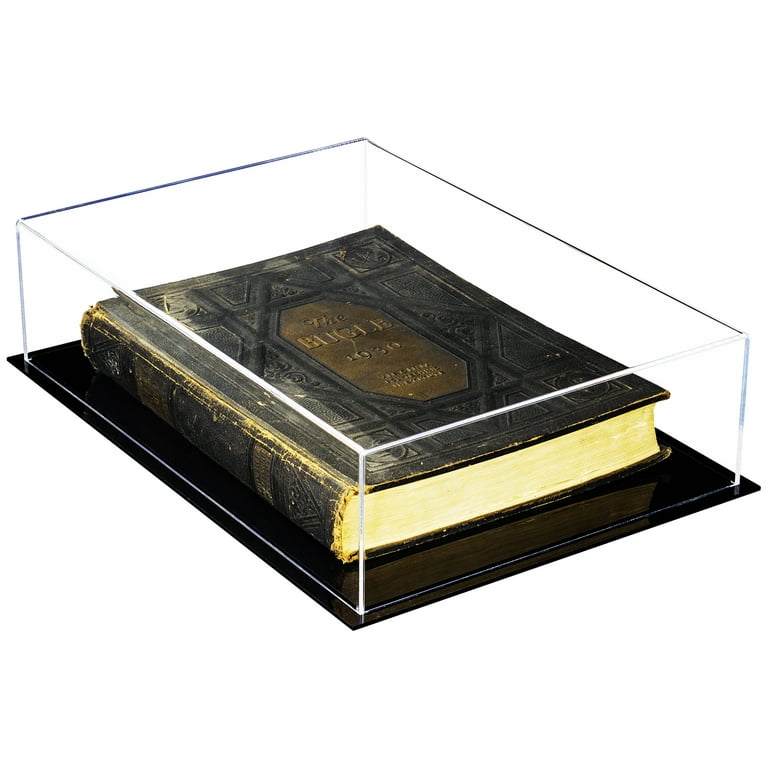The image features an old leather-bound book titled "The Bugle 1930," encased in a clear protective display case. The book is positioned slightly tilted to the left, almost at a 45-degree angle, resting on a solid black base, which could be made of either plastic or marble. The book's cover is predominantly black with intricate embossed and embellished designs, and it shows significant signs of aging with noticeable scrapings and discoloration along the edges. The title and year, "The Bugle 1930," are prominently displayed in an oval-shaped brown area on the front cover. The entire setup is centered against a stark white background, emphasizing the book as the focal point. The glass case encases the book from all sides, ensuring its protection and adding to the display's elegance.